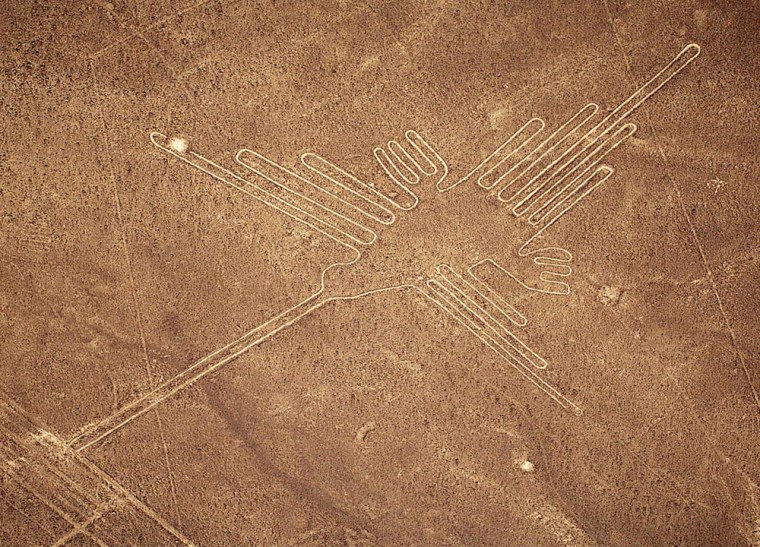This image captures an aerial view of the Nazca Lines, specifically depicting a bird etched into the brown, barren terrain. The figure of the bird is intricately designed with numerous elongated lines and shapes representing various parts of its body. The head, slightly round with an extended beak, seamlessly transitions into a series of ovals and curved rectangular shapes that form the wings. Each wing exhibits multiple straight lines that extend outward, with the longest line being about twice the length of the shortest. The overall design is meticulous and appears as a graphic representation of a bird, almost like a hieroglyphic. The background is largely dirt, with spots of vegetation, and the ground seems darker towards the edges of the image. The lines are precisely drawn, suggesting they were carefully created from an elevated perspective.